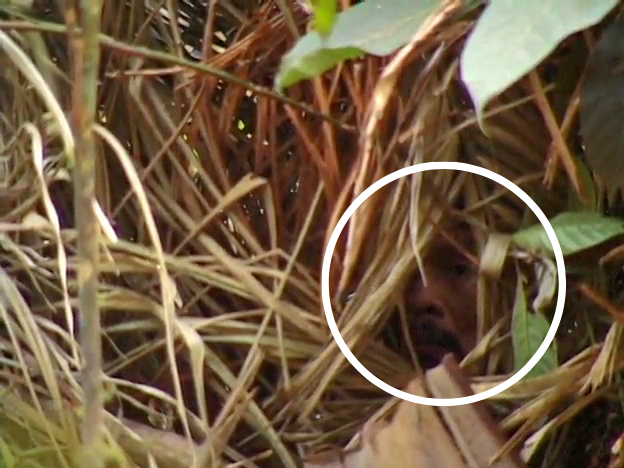This detailed photograph captures an outdoor scene in a dense, jungle-like field during daylight. The area is thick with criss-crossing dry, reedy brown branches and some patches of green leaves, giving an impression of an intricate and somewhat chaotic thicket. A few elongated green leaves dangle from the upper right corner, adding a splash of color amidst the predominantly dry foliage. Notably, a vivid white circle is drawn on the lower right-hand side of the image, which draws the viewer's focus to a hidden face within the brush.

Peering through the tangled branches, the circled area reveals a man of Asian descent with light brown skin. Only the left side of his face is visible, including his brown eye, short domed nose, a black mustache, and full lips. His expression appears soulful and wary, enhancing the ominous and watchful mood of the scene. Sunlight filters from above, illuminating parts of the foliage and adding depth to the mysterious ambiance. The white circle around the man's face is crucial, as it helps to pinpoint his hidden yet alert presence amidst the seemingly impenetrable undergrowth.